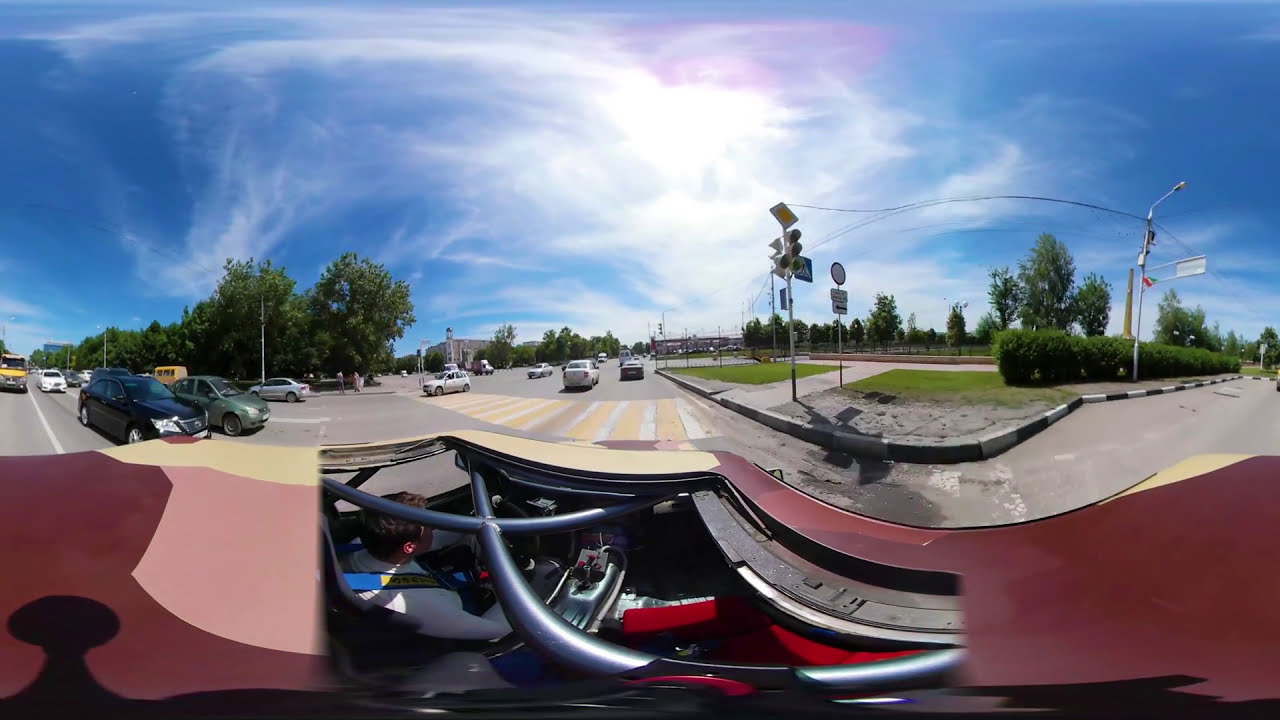The outdoor daytime city street scene is dynamic and distorted due to the wide-angle lens, capturing a bustling intersection from an elevated car perspective. A man in a white T-shirt drives the car, visible through what appears to be an open sunroof or from a dash cam. His vehicle, a brownish-maroon car, is surrounded by various cars—silver, white, green, and black—on a street with a mix of cars traveling in different directions. The intersection features multiple traffic elements including an unreadable street sign on the left, a traffic light with a diamond sign at the corner, and another circular sign. The crosswalk below, painted in yellow and white, stands out prominently. The right side of the street shows a serene strip with greenery, bushes, trees, and possibly a park area. Despite the high white clouds giving a hint of overcast, the sky is predominantly blue, making the scene lively and vivid. Silver-colored cables, possibly power lines, run throughout the setting, and although there are designated sidewalks with ample greenery, no pedestrians are present, contributing to the modern urban feel of this street corner.